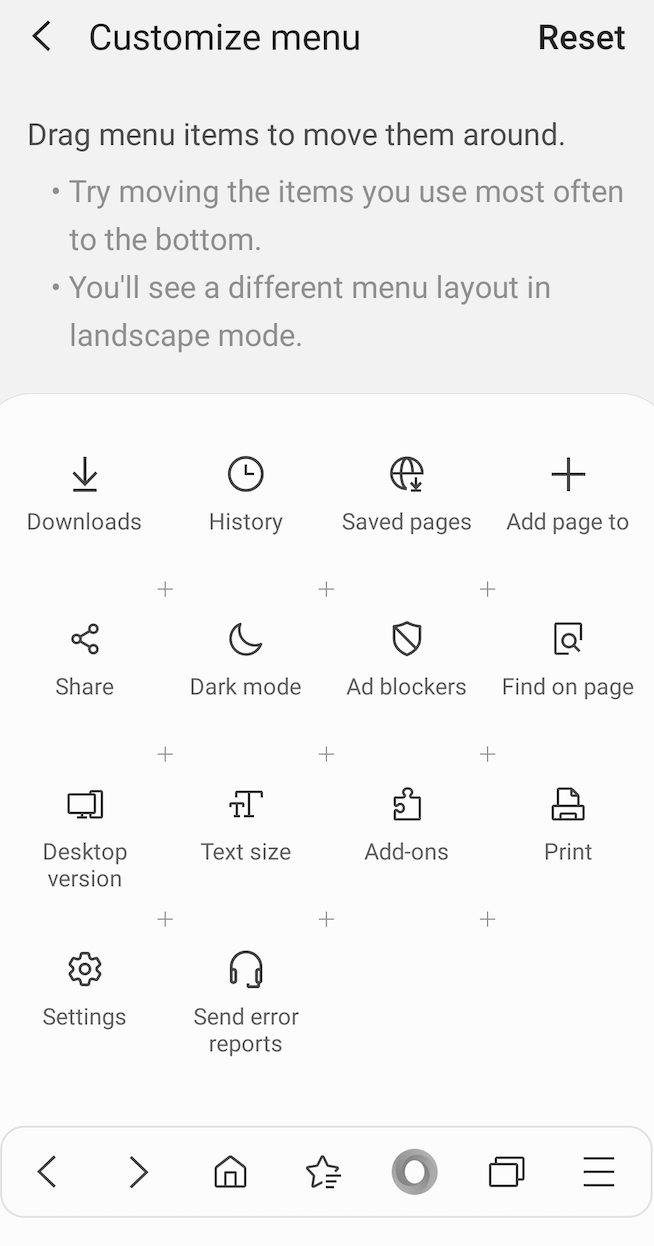The image appears to be a screenshot taken from a mobile phone screen, featuring a customizable menu interface on a white and gray background. The upper part of the screenshot displays a gray box. In the upper left-hand corner of this box, there is a black arrow pointing to the left with the text "Customize Menu" next to it, both words capitalized. On the right side of the gray box, the word "Reset" with a capital 'R' is displayed. Below this gray header, there is an instructional text that reads, "Drag menu items to move them around. Try moving the items you use most often to the bottom. You'll see a different menu layout in landscape mode."

Beneath the instruction, various icons are organized into four rows, each with corresponding labels:

1. **First Row (left to right)**:
   - **Downloaded Arrow**: Labelled "Downloads".
   - **Clock Icon**: Labelled "History".
   - **Globe with Downward Arrow**: Labelled "Save Pages".
   - **Plus Icon**: Labelled "Add Page To".

2. **Second Row (left to right)**:
   - **Three Circles Linked by Lines** (resembling a sideways 'V'): Labelled "Share".
   - **Crescent Moon Icon**: Labelled "Dark Mode".
   - **Shield with Diagonal Stripe**: Labelled "Add Blockers".
   - **Square with Magnifying Glass**: Labelled "Find On Page".

3. **Third Row (left to right)**:
   - **Old Large Computer Monitor**: Labelled "Desktop Version".
   - **Small and Large T (different text sizes)**: Labelled "Text Size".
   - **Puzzle Piece Icon**: Labelled "Add-Ons".
   - **Printer Icon**: Labelled "Print".

4. **Fourth Row**:
   - **Gear Icon**: Labelled "Settings".
   - **Headphones Icon**: Labelled "Send Error Reports".

At the bottom of the image is a rectangular section with a series of navigation icons:
   - Arrow pointing left.
   - Arrow pointing right.
   - Home icon.
   - Star with three lines.
   - Circular lens.
   - Two-panel squares.
   - Three stacked horizontal lines.

This detailed description captures each element of the menu interface, specifying the icons and their labels for a comprehensive understanding of the layout.